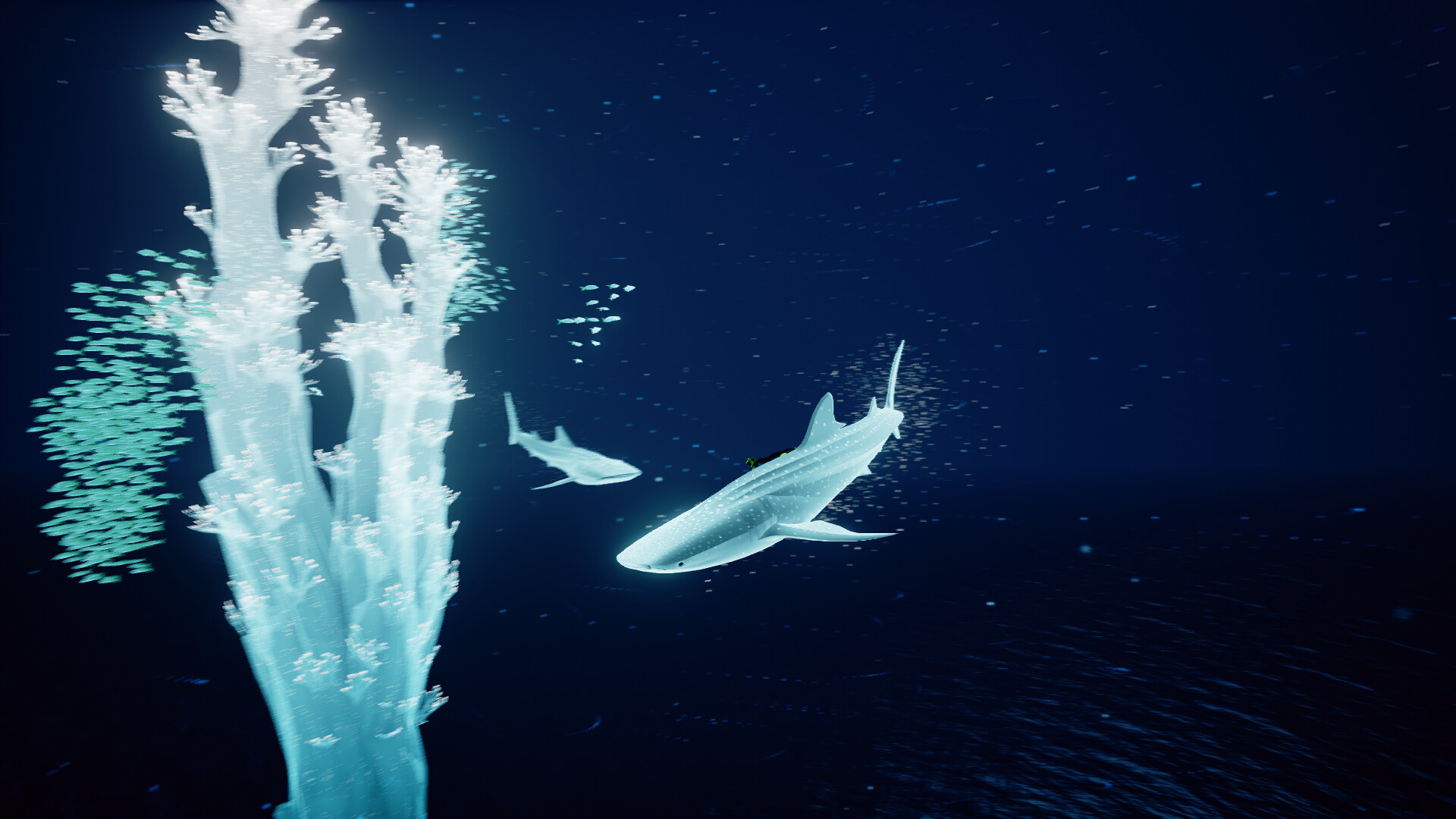The image appears to be a digitally rendered or animated underwater scene, blending elements of marine life with celestial motifs. Dominating the left side of the scene is a large piece of coral, depicted in blue with delicate, white fiber-like extensions. Surrounding the coral are tiny, light turquoise specks, resembling schools of fish swimming amidst the dark blue ocean background, which is dotted with light blue circles, evoking the appearance of air or water bubbles. The darkness intensifies towards the bottom, particularly on the left, while the right side shifts to a lighter hue. 

Interspersed throughout the scene are what appear to be small fish, shifting towards the left, with more visible on the right side of the coral. In the foreground, there are two sharks, one drawn in a light blue-gray color and the other positioned perpendicular to it, both featuring distinct tails and rounded noses, reminiscent of hammerheads. The background, transitioning from deep ocean blues to lighter tones at the horizon, displays numerous white speckles that suggest either underwater particles or perhaps stars, giving the impression of a night ocean scene blending with a starry sky. Overall, the image uniquely combines underwater features with an ethereal, almost celestial environment.